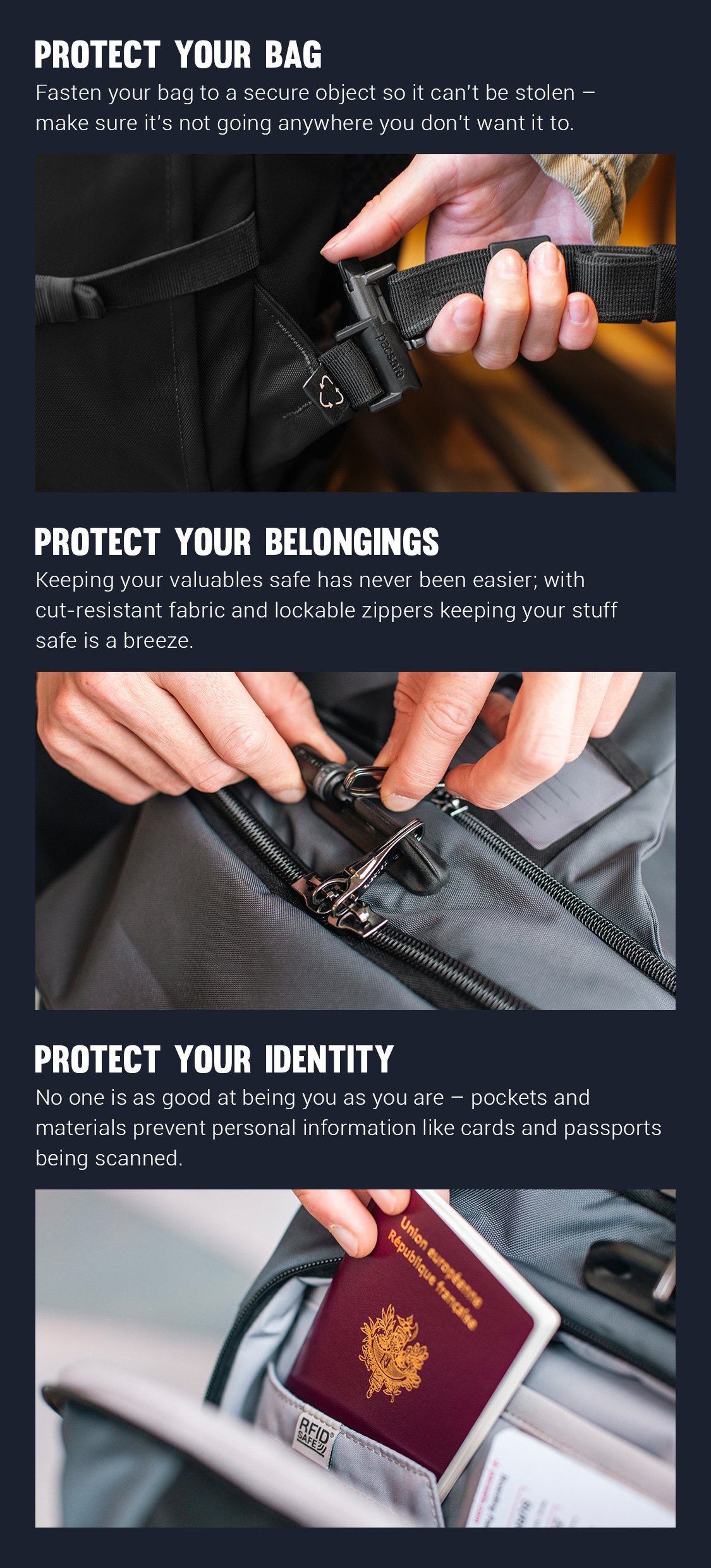The poster features three sections, each with images and white text on a vertical rectangle with a gray transitioning background. The top section, titled "PROTECT YOUR BAG," displays a large capitalized heading with a brief description below, next to an image of a person's hand securing a bag strap. The middle section, labeled "PROTECT YOUR BELONGINGS," includes a heading in large white letters, followed by a short descriptive paragraph and an image of hands locking a bag zipper. The bottom section, titled "PROTECT YOUR IDENTITY," also in bold white letters, contains a concise explanation below the heading, accompanied by an image of fingers inserting a passport into a secure pocket. The poster provides comprehensive tips for securing bags with cut-resistant fabric and lockable zippers, and using materials that prevent unauthorized scanning of personal information, such as cards or passports.